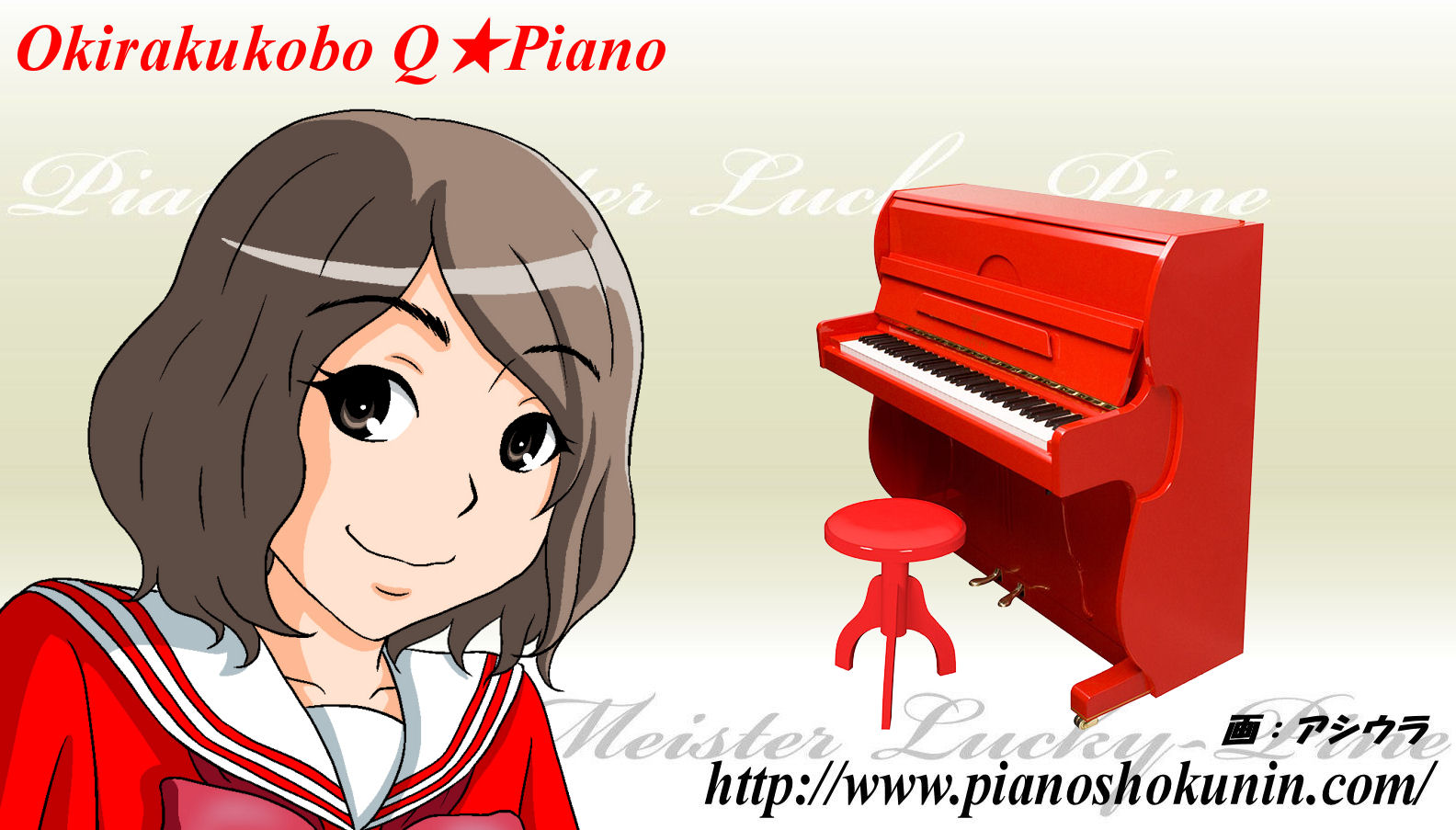The image appears to be an animated advertisement for a red piano. On the left side, there is a cartoon-like drawing of a young girl with brown hair. She is wearing a red sailor-type top with a white collar and underneath, a white shirt. The girl has a half-smile and is looking straight ahead. Behind her, partially obscured by her figure, are some white text elements, one of which reads "piano." Above her, in the upper left corner, the text "Okurakukobo Q" is displayed alongside a red star and the word "Piano."

On the right side of the image is a bright red upright piano with black and white keys. Accompanying the piano is a shiny red stool positioned in front of it. The background features a brown and white pattern with more obscured white text, including the words "Meister Lucky" in the lower right corner. Further down in the bottom right is a black text providing a website URL: "http://www.pianoashokunin.com."